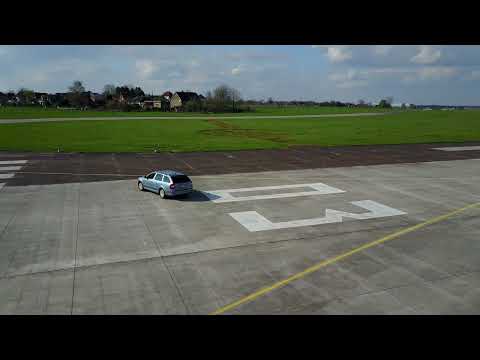This drone photograph, characterized by its realist style and landscape orientation, captures a top-down view of a vast gray concrete slab, which resembles an airplane tarmac or a helicopter landing pad. Centered in the image is a light blue, four-door station wagon, possibly a Mercedes-Benz, parked on the expansive surface. The concrete area is marked with a large, white number "03" and features a yellow stripe that curves from the bottom left corner of the image toward the "03" before straightening out. Beyond the car, the photograph reveals a lush, bright green grassy field, leading to a distant, sizeable farmhouse amidst other houses and a road. The scene extends into a blue sky dotted with white clouds, framed by horizontal bands of black at the top and bottom of the image, emphasizing the vastness and clarity of the open space.